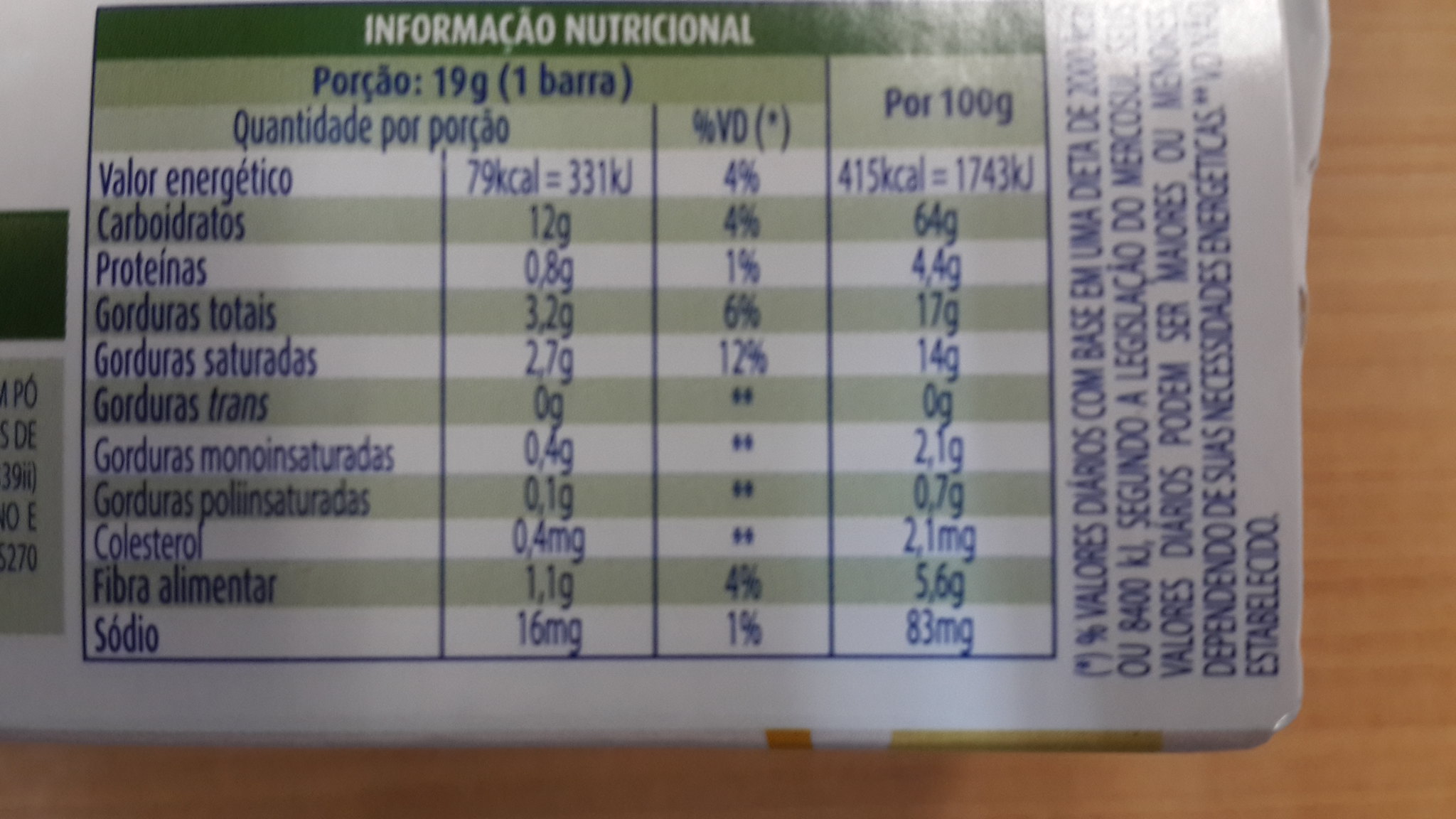This photograph showcases the nutritional information on a food package, set against a blonde, vinyl wood-like surface. The nutritional table itself features horizontal stripes in varying shades of green, reminiscent of celery stalks, transitioning from dark green to light green and finally to white. The information is presented in a bold blue font. The table is divided into four columns: the first listing the ingredients in Spanish, the second detailing the number of grams, the third indicating the percentages, and the fourth showing the total grams per 100 grams. On the right side of the image, oriented differently than the main table, the ingredients are once again listed in Spanish.